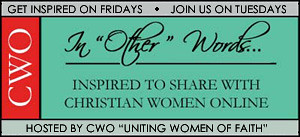The image is a rectangular flyer or poster with a black border at the very top. Beneath this, a thin horizontal gray line holds the text, "Get inspired on Fridays, join us on Tuesdays," in black letters. Along the left-hand side, a red vertical rectangle with large white letters displays "CWO." Directly under the initial gray line, a green rectangular box appears, containing the italicized text, "In other words," followed by an underline. Below this tagline, in a serif font (likely Garamond), it states, "Inspired to share with Christian women online." The lower section of the flyer features another thin gray strip with the text, "Hosted by CWO, Uniting Women of Faith," in a sans-serif font. The entire poster has a clean, teal-colored background that emphasizes the text and design elements effectively.